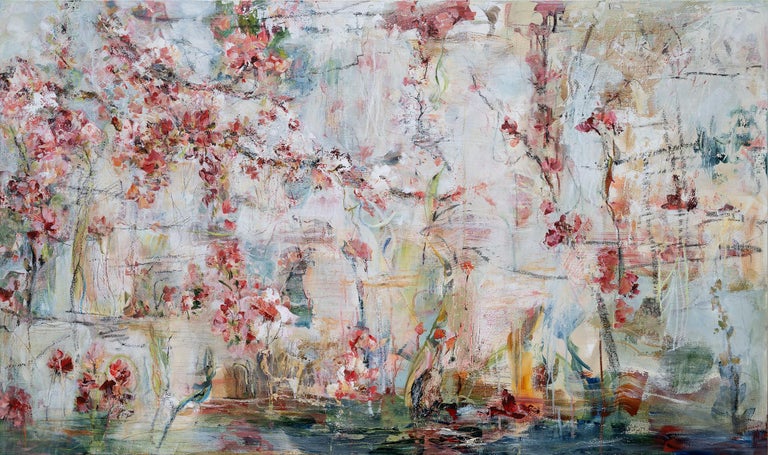The rectangular painting, with its delicate pastel color scheme ranging from light pink to green and yellow, evokes the ethereal quality of watercolor art, though it may also suggest crayon with faint, scratchy marks scattered throughout the composition. At first glance, the painting's minimalist, abstract approach leaves much to the imagination. The most prominent feature is a backdrop of gray that supports an array of flowers, predominantly in shades of pink, red, and orange, which seem to float above a nondescript, almost spectral outline that might suggest branches, vines, or even figures and boats.

These floral forms, indefinite in their detail, hint at cherry blossoms, dogwoods, or roses, with the difficulties in making out clear shapes adding to its abstract allure. Below, in the bottom-right corner, there appears to be a pool of water with what seems to be lily pads, adding another layer of complexity to the scene. The interplay of light and dark versions of the pinks and greens coupled with the stylistic ambiguity gives the artwork an impressionistic feel, making it well-suited for an exhibit in a modern art museum.